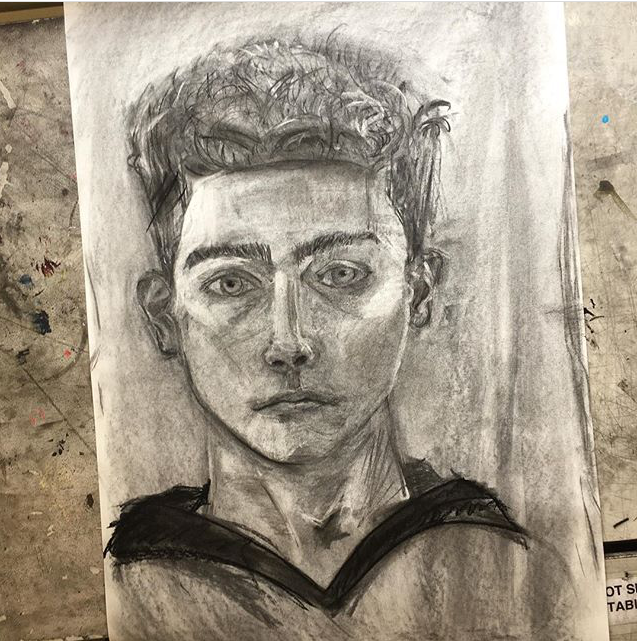This is a meticulously crafted pencil or charcoal drawing of a young boy on a white canvas or paper. The boy’s hairstyle is distinctive, with closely trimmed sides and a voluminous, puffy top. He is depicted wearing a hoodie, which adds a casual and contemporary touch to the portrait. The artist has painstakingly detailed his facial features, which include well-defined eyebrows, expressive eyes, a nose with distinct nostrils, and full lips. His ears are symmetrically placed, framing his face that also features prominent cheekbones, a defined chin, and a strong jawline. The neck showcases subtle anatomical details like the jugular vein and Adam's apple. The intricate rendering extends to the general structure of the boy’s skull and eye sockets, demonstrating an impressive understanding of human anatomy. The background of the drawing has a gray, slightly textured appearance, which contrasts beautifully with the white canvas and gives the image a sense of depth and dimension.